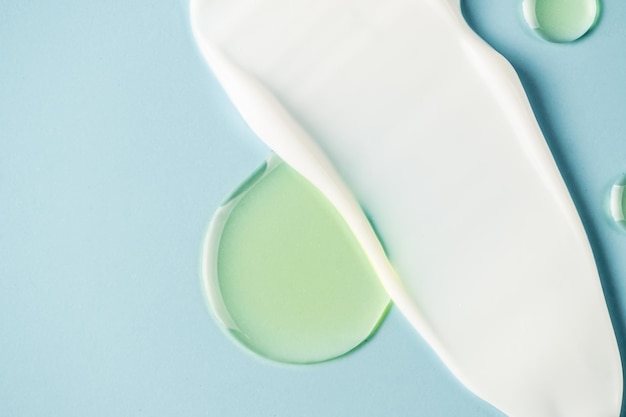This close-up landscape photograph captures a light pale blue surface, possibly a table, with various blobs of paint or a waxy substance scattered across it. At the center of the image is a thick, circular green substance, surrounded by white edges, giving it a waxy or resin-like appearance. From the top center, a large, thick white streak of the same waxy consistency meanders diagonally down to the bottom right, dominating the frame. In the upper right corner, two smaller green circles are partially visible, with one nearly cut off at the top and the other along the middle right edge. The scene is devoid of any people or text, focusing solely on the abstract interplay of the green and white waxy substances against the serene blue background.